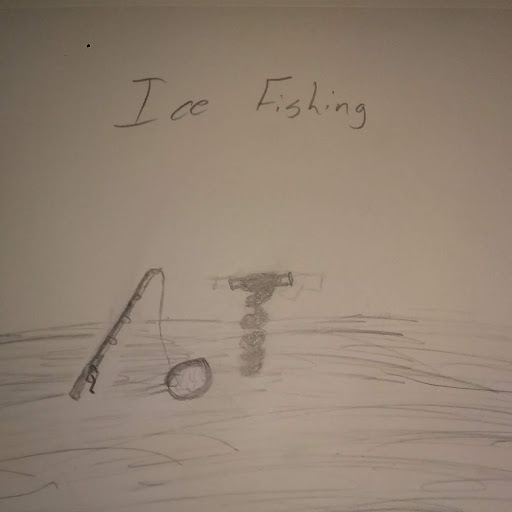The image is a photograph of a simple pencil drawing on plain white paper. At the top of the drawing, the words "Ice Fishing" are written in pencil with the letters "I" and "F" capitalized. About one-third down the page, a simple horizon line is drawn, with minimal shading to represent the ground or ice surface. In the center of the image, a fishing rod and reel are propped up on a stand with a fishing line extending downward into a hole, presumably an ice fishing hole. Next to the fishing setup, there is a crudely drawn object resembling a corkscrew or wine opener, likely intended to represent a tool used to create the hole in the ice. The background is otherwise plain, emphasizing the simplicity of the landscape and the central elements of the drawing.